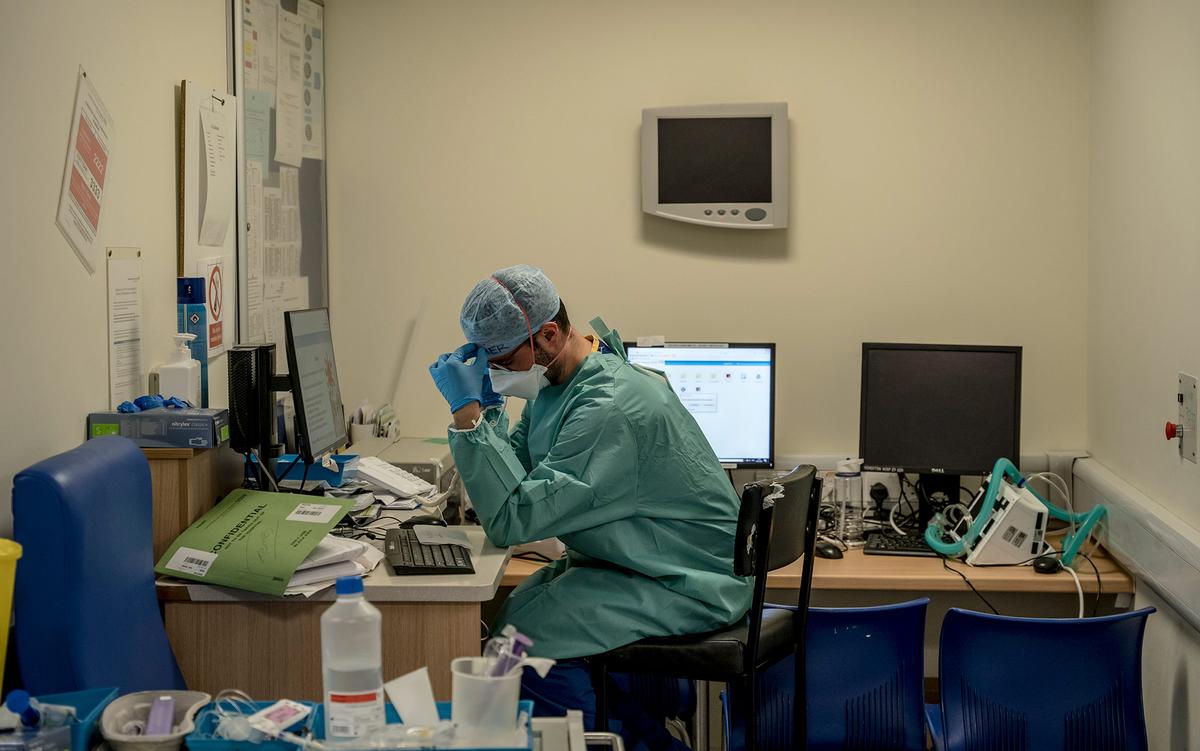This photograph captures a moment inside a cluttered and chaotic doctor's office, where a surgeon, fully dressed in green surgical attire and blue scrubs, sits at a desk appearing deeply disturbed or in contemplation. He rests his left hand on his forehead while looking down at a piece of paper placed on a black keyboard. The desk is extremely busy, strewn with folders, medical equipment, and charts. Surrounding him are three computer screens, one of which he faces, and a wall-mounted monitor. A bulletin board and wall behind are densely covered with charts and papers. In the foreground, there is a table displaying medical supplies like bottles, basins, and wipes. Additionally, a machine with green tubes lies next to an unused computer, and the overall scene exudes a sense of disarray and frustration, contributing to the doctor's evident stress.